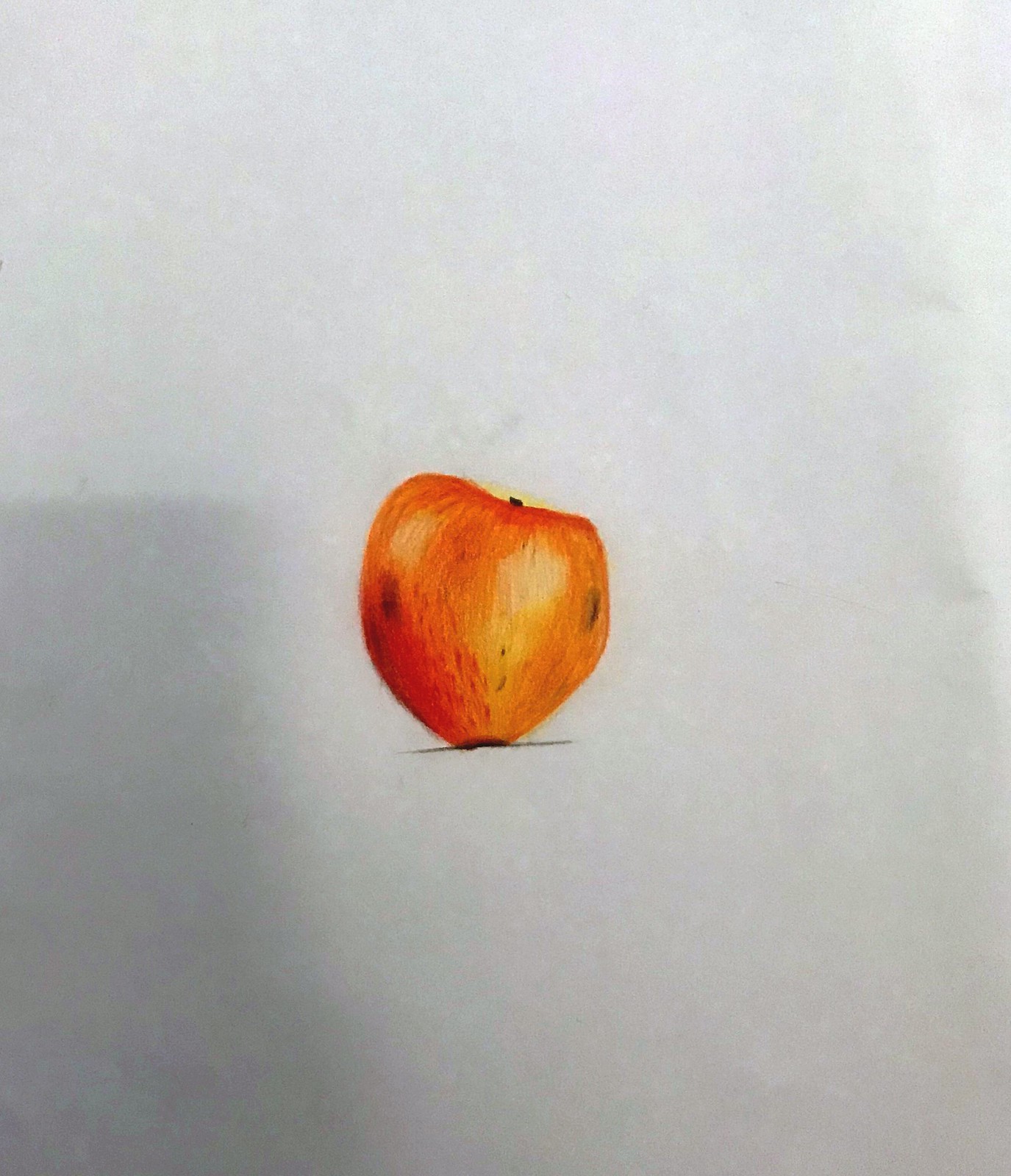This image showcases a detailed and colorful pencil drawing of an apple, carefully rendered on paper. The apple, occupying a central placement within the composition, is accentuated in vibrant hues, skillfully brought to life using colored pencils. It exhibits an irregular, lopsided shape, with the left side evidently fuller than the right. 

The artist has masterfully blended multiple shades of orange, red, brown, and yellow to create a realistic texture that enhances the apple's visual appeal. A delicate, black shadow is subtly cast beneath the apple, grounding it on the white paper surface, while a slender black stem protrudes from the top, adding to the natural appearance of the fruit. 

Distinctively, the apple features two prominent black spots, each situated on either side, amidst various darker textured markings that further contribute to its detailed and lifelike representation.